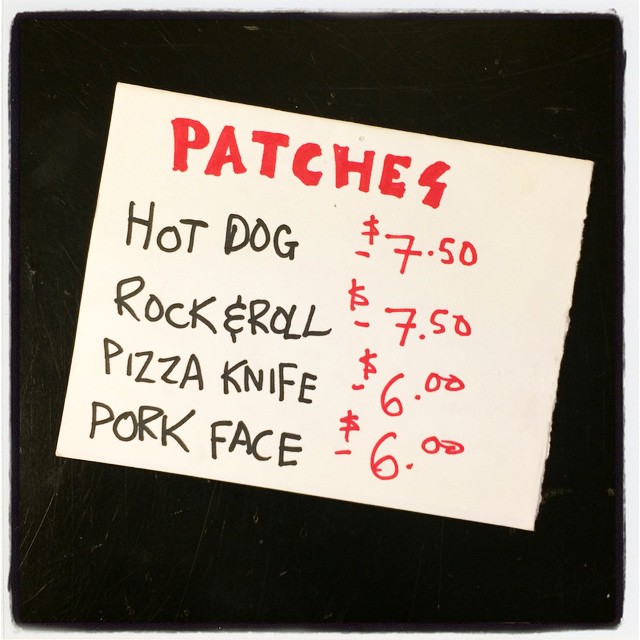The image shows a black background featuring a single, slanted white paper in the center. At the top, in bold and capitalized red letters, it says "PATCHES." Below this, the menu lists four items in black text on the left, each followed by their price in red text on the right. The items are: "HOT DOG" priced at $7.50, "ROCK & ROLL" also priced at $7.50, "PIZZA KNIFE" at $6.00, and "PORK FACE" at $6.00. A small hyphen separates each item from its cost. The overall layout appears handwritten, adding a personalized touch to the presentation.